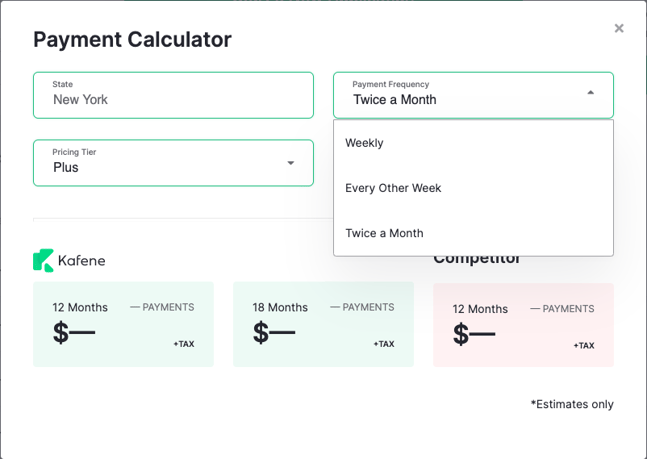The image features a payment calculator interface set against a white background. On the left-hand side, the title "Payment Calculator" is prominently displayed in large black letters. Below this title, there are several interactive fields and options.

Firstly, there is a green box labeled "State," where "New York" has been entered as an example. Adjacent to this box is another green box labeled "Payment Frequency," which includes a dropdown menu. The selected option is "Twice a month," but other available choices include "Weekly" and "Every other week."

Beneath the "State" field, there is a dropdown menu labeled "Pricing Tier" where "Plus" has been selected. In the central section of the interface, the name "Kafene" is displayed in capital letters (K-A-F-E-N-E), accompanied by a green and white icon, presumably representing the company.

Below this central section, there are three boxes, each offering different payment plans:
1. The first box is gray and indicates "12 months payments," with a dollar sign and a small "plus tax" notice in the lower right-hand corner.
2. The second box offers an "18 months payment" plan, with a prominent dollar sign in the lower right-hand corner.
3. The third box is pink and also mentions "12 months payments," featuring a dollar sign and "plus tax" with an asterisk. The asterisk denotes that the amounts are "estimates only."

Overall, the interface is clean and user-friendly, designed to guide users through each decision step by step effectively.